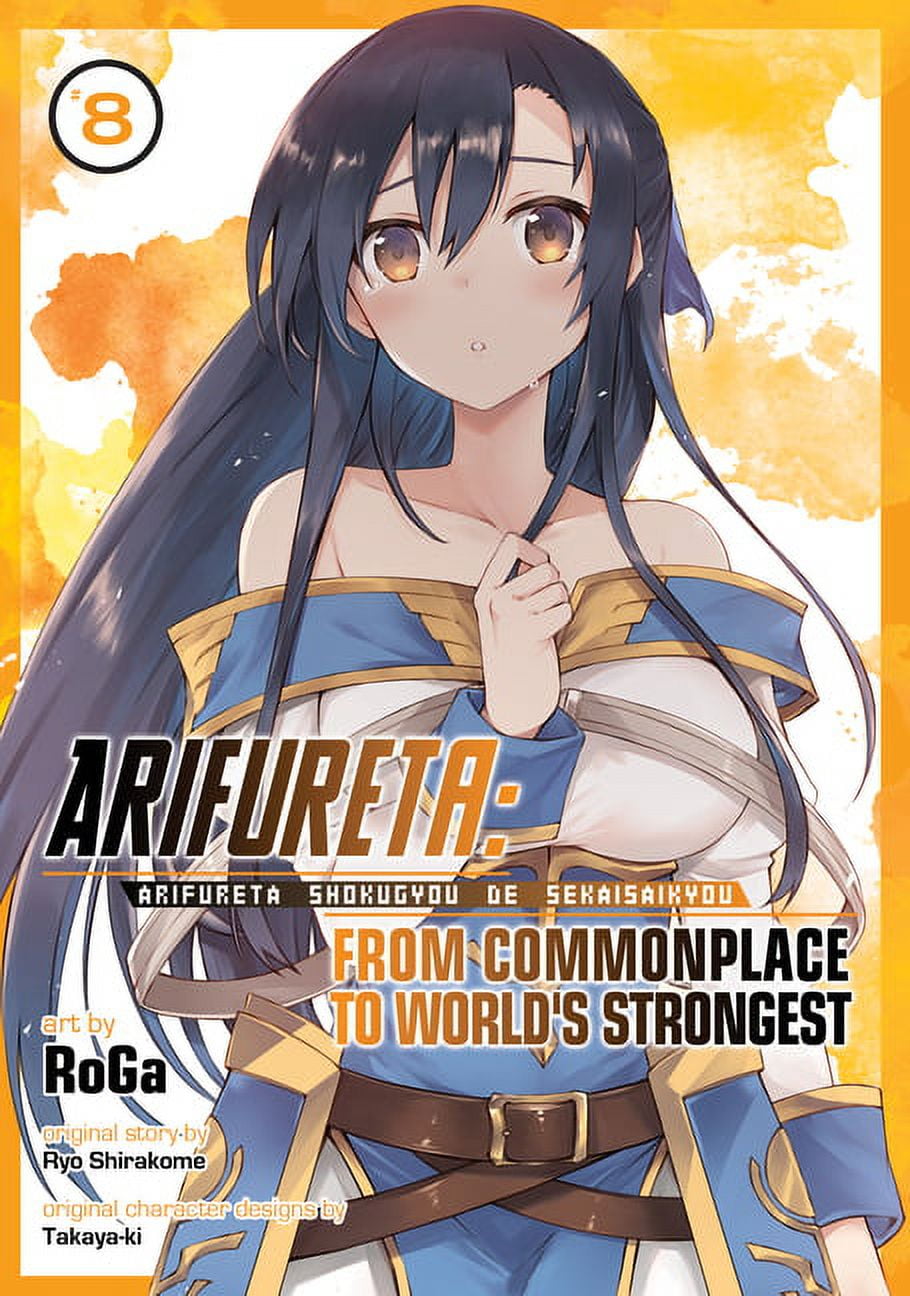The image features an eye-catching magazine cover set against an orange and white background, framed by a distinct orange border. In the top left corner, the number "8" appears within an orange circle on a white background, likely indicating the magazine's edition number. Dominating the cover is an anime-style illustration of a female character named Arifureta, from "From Commonplace to World's Strongest." She appears striking with her long, flowing hair that transitions from black to purple with hints of blue hues, and expressive purple and gold eyes. She is attired in a strapless top, with additional details including a brown belt and golden blue cuffs. At the bottom left, credits are given for the artwork and story: "Art by Roga," "Original Story by Ryo Shirakami," and "Original Character Design by Takaya Ki." This vividly detailed cover showcases a vibrant piece of anime artwork, potentially for a gaming magazine.